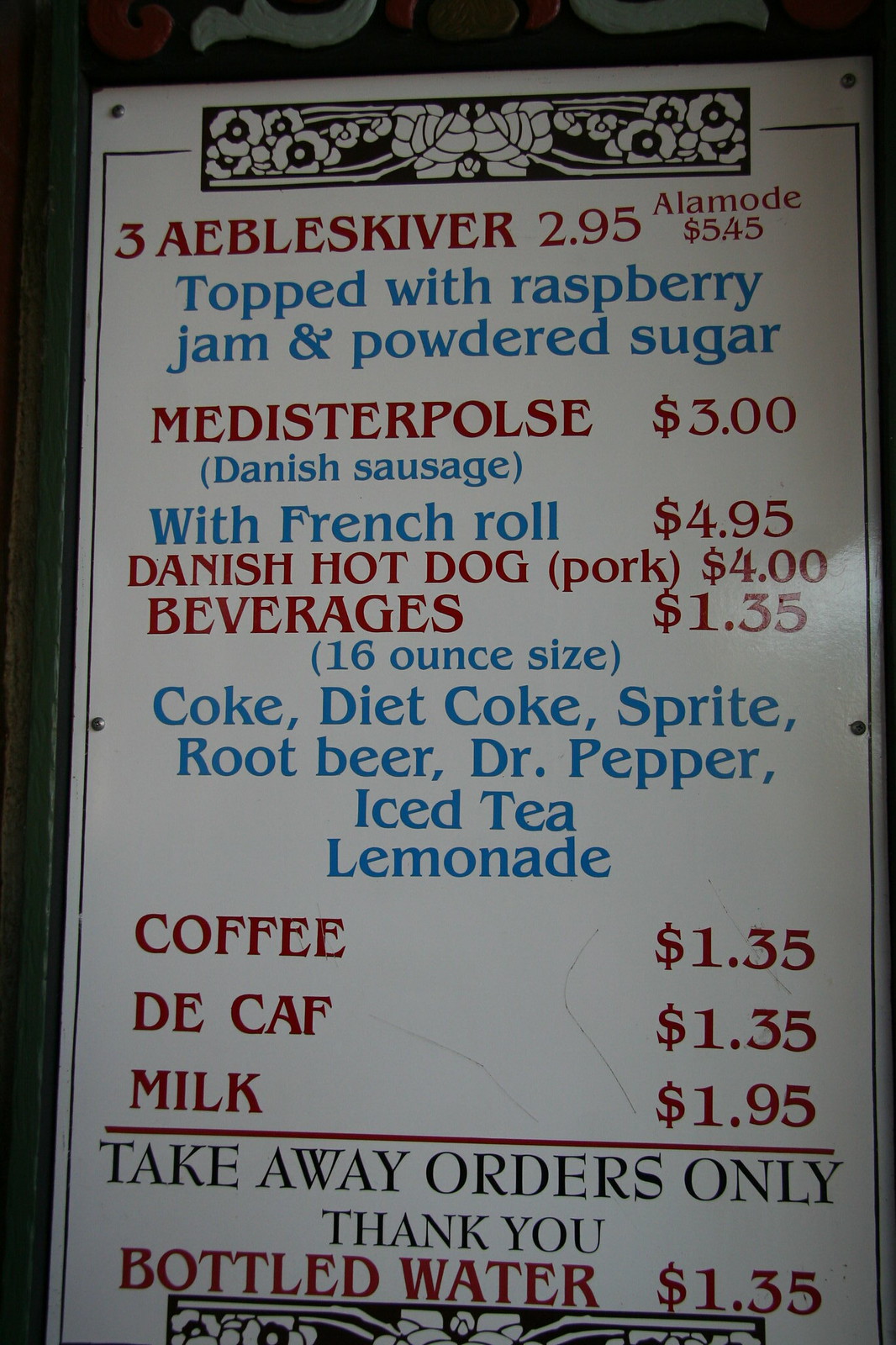The image depicts a menu displayed on a sign that resembles a whiteboard. The text on the menu is typed, not handwritten. At the top of the sign, there is a small black illustration of a floral pattern. Below this, bordered in black, the menu items are listed:

- **3 Ableskiver**: $2.95  
  - **A la Mode**: $5.45  
  - Both prices are marked in red with a vertical line extending from the bottom of the dollar sign.
  - Description (in blue): Topped with raspberry jam and powdered sugar.

- **Metastere Pulse**: $3.00
- **Danish Sausage (with French roll)**: $4.95
- **Danish Hot Dog** (Pork): $4.00

Beverages, listed in a single column with a size specification of 16 ounces, include:
- **Coke**: $1.35
- **Diet Coke**: $1.35
- **Sprite**: $1.35
- **Root Beer**: $1.35
- **Dr. Pepper**: $1.35
- **Iced Tea Lemonade**: $1.35
- **Coffee**: $1.35
- **Decaf**: $1.35
- **Milk**: $1.95

A red line separates these items from a note stating, "Takeaway Orders Only. Thank You."

- **Bottled Water**: $1.35

At the bottom of the sign, another black floral pattern illustration mirrors the one at the top.